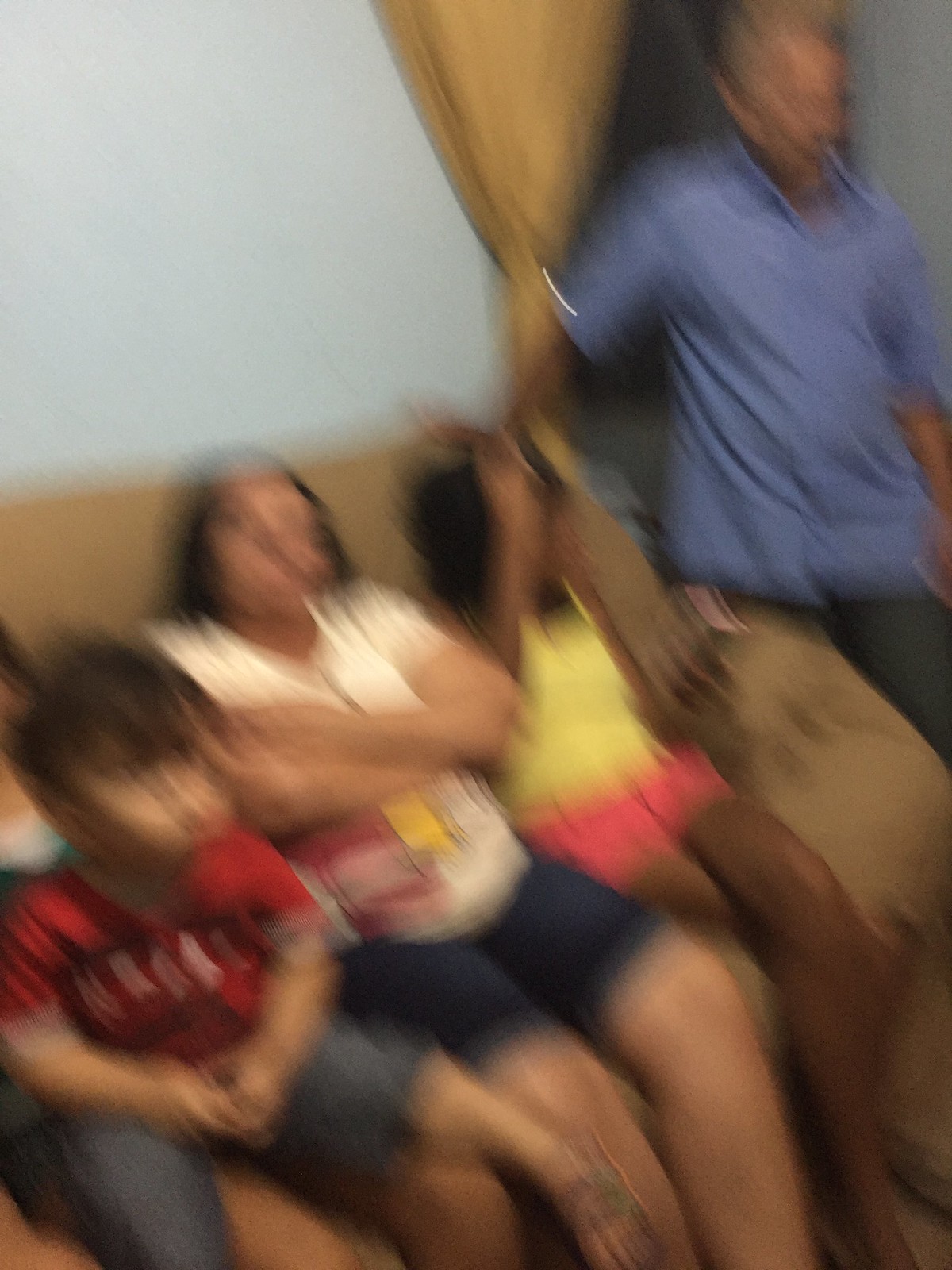In the image, a family is gathered around on a tan couch with tan drapes in the background. At the center of the couch sits a woman wearing black shorts and a cream-colored shirt adorned with a mixture of red, yellow, and white designs. She has brown hair, folded arms, and is looking directly into the camera. To her right is a little boy with brown hair, dressed in a red shirt and jeans, who is gazing off to the side. Directly behind him, partially obscured, is another child with black hair, identifiable by a turquoise garment and a visible leg. To the woman's left sits a girl with black hair, wearing a yellow top and red shorts. Standing beside her is a man dressed in a short-sleeved blue collared button-down shirt and dark pants, slightly looking down at the floor. The family appears relaxed and comfortable in their living space, which features a white wall beyond the couch.